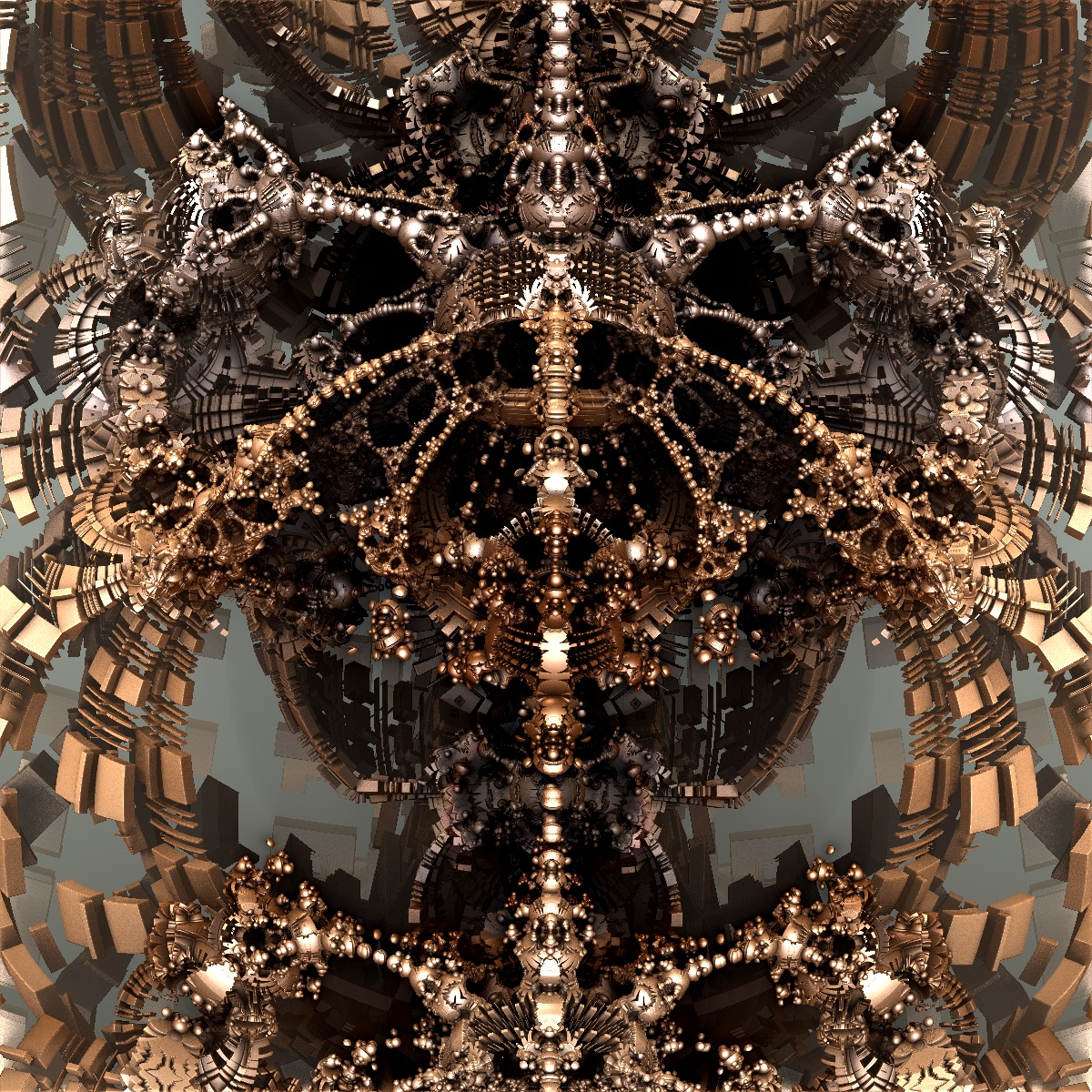The image depicts a highly detailed 3D fractal art piece that resembles a chandelier, viewed from beneath and looking up into the ceiling. The primary focus lies in the center of the composition, featuring a central elliptical hub adorned with ornate: silver arms extending upwards and gold arms extending downwards. There is a prominent vertical structure, filled with reflective knobs and circles, which creates a complex interplay of reflections and metallic surfaces. The background is a dark area filled with abstract, floating squares in shades of light grayish blue, lending a sense of depth and dimension. The overall color palette includes various metallic tones such as silver, gold, copper, as well as hues of black, tan, beige, chocolate, and light yellowish white. The lower half of the image appears somewhat less clear, as if reflected on a glass surface. The entire scene is set against an empty, blue-tinged backdrop, adding to the surreal and abstract nature of the artwork.